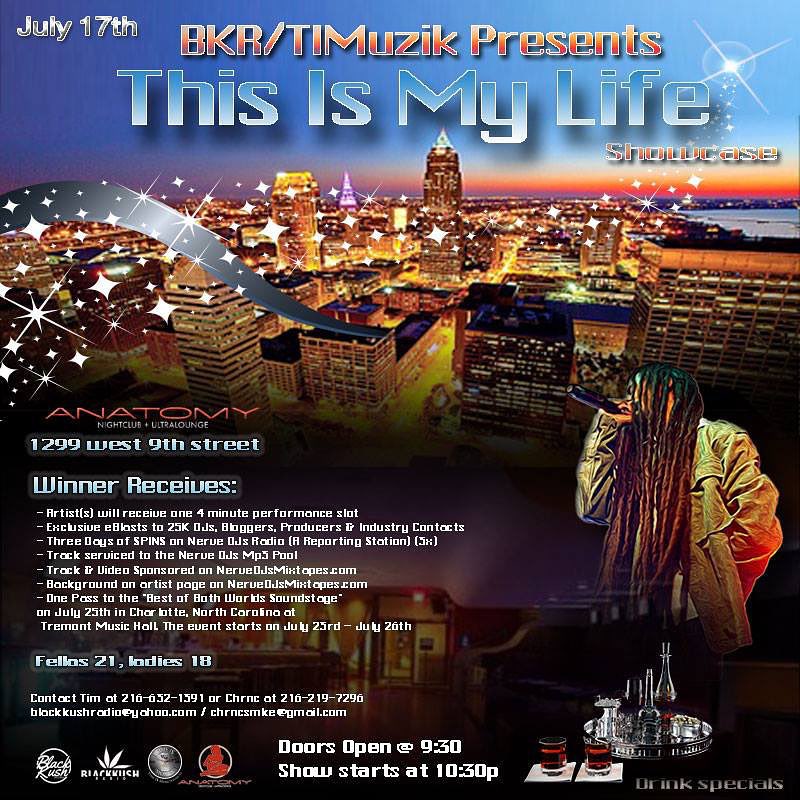The detailed caption for the image is as follows:

This vibrant poster, promoting an event on July 17th, is a mixed collage of colorful and dynamic elements. The top portion, dominated by the headline "BKR/TM Music Presents: This Is My Life Showcase," features a cityscape at night, bathed in warm orangey-brown illumination and adorned with twinkling stars. A noticeable sunset casts a picturesque backdrop over the urban skyline. On the middle right, a person with long, flowing black dreadlocks is passionately singing into a microphone, directed towards the nine o'clock position. Below this figure, there's a tray garnished with a carafe of red wine, accompanied by two glasses placed on white napkins. The lower left quadrant lists enticing prizes for contest winners and includes detailed event information, such as the venue "Anatomy Nightclub" at "1299 West 9th Street." The event stipulates that "fellas must be 21" and "ladies 18" years of age. Contact details and several logos, including one featuring a marijuana leaf, embellish this informational section. The center bottom prominently notes "doors open at 9:30 PM" and "show starts at 10:30 PM."